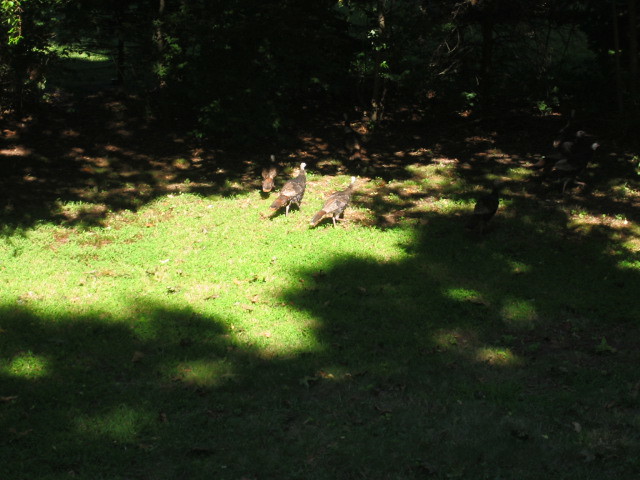The photograph captures a scene in a natural, wooded area on a sunny day. The image predominantly features deep shadows, both at the top and the bottom, framed by dark silhouettes of trees. Only a small patch in the center-left of the picture is illuminated by sunlight, revealing a grassy ground that hints at spring or summer. In this sunlit area, three large brown birds, possibly turkeys or pheasants, are seen walking rather than flying. The birds are facing away from the photographer, their heads slightly visible but blurred, making identification challenging. Their bodies are adorned with brown feathers, and they have distinct brown tail feathers. The overall blurriness of the photo adds to the difficulty in discerning finer details, but the ambiance of the shaded woodland with a burst of light in the center is clearly captured.